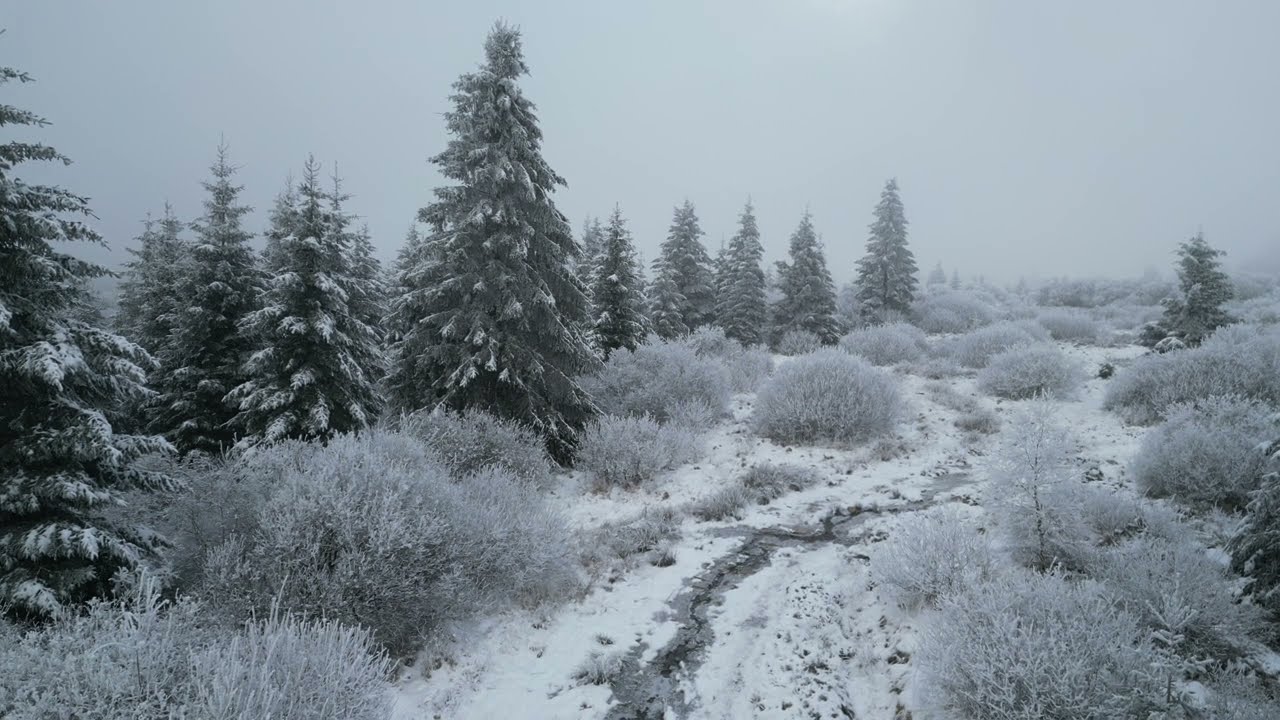The photograph captures a serene, wintry landscape in a mountain region immediately after snowfall. The scene is dominated by a gray, overcast sky that casts a muted tone over the entire image. In the foreground, a winding dirt path, flanked by low, round bushes heavily blanketed in snow, leads from the center bottom towards the upper right of the photograph. To the left of the path, a dense cluster of approximately 10-12 pine trees stands tall, their needles dusted with fresh snow. The right side of the image features mainly snow-covered bushes, with a single pine tree visible at the top right. The terrain suggests a remote, deserted area, devoid of any human presence or structures, emphasizing the untouched beauty of the snow-laden wilderness.